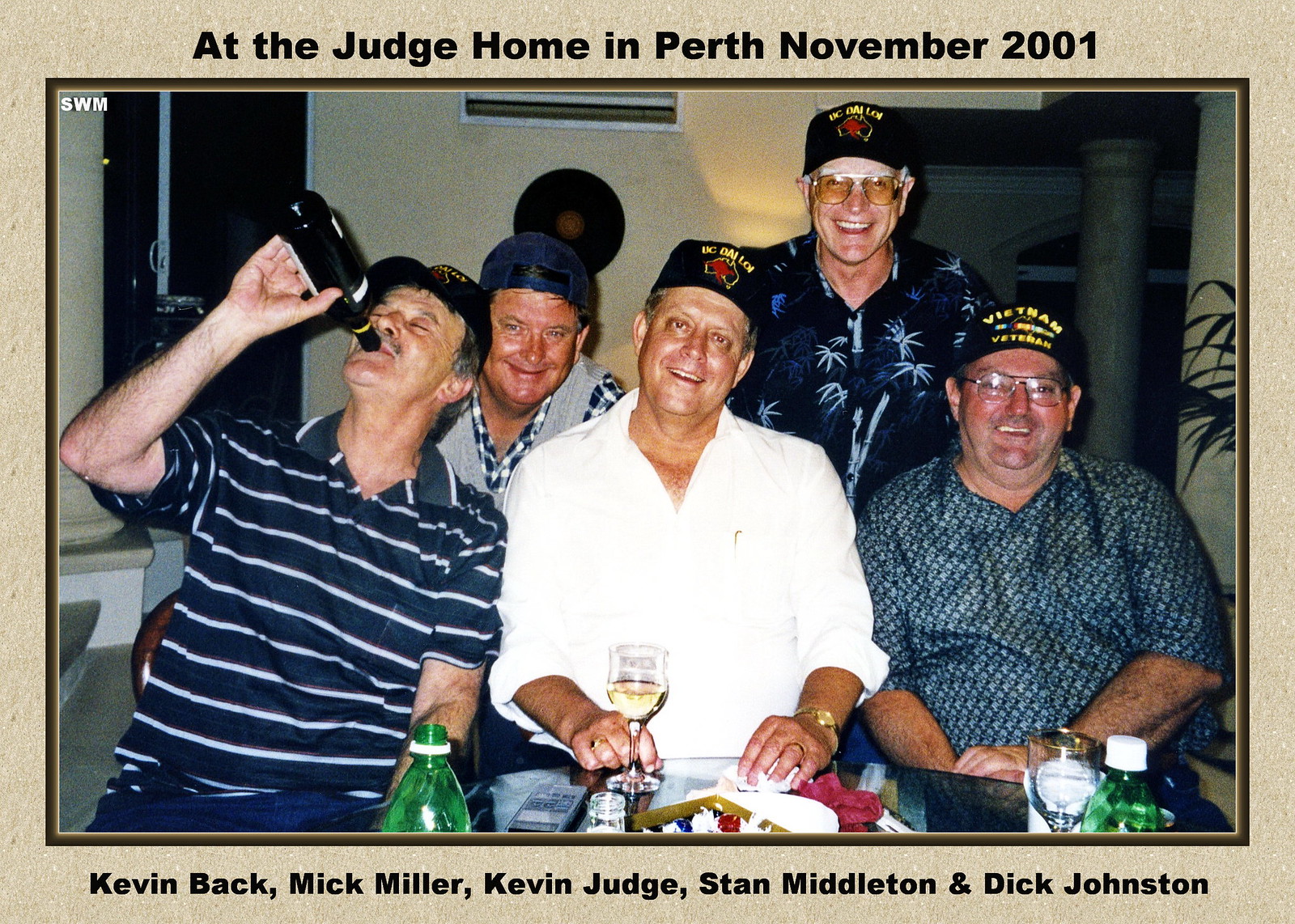The image features a photograph of five men gathered around a clear table adorned with soda bottles and wine glasses. The photograph is bordered by a light tan frame with a dark brown inner border. The top of the tan border bears black text reading, "At the Judge Home in Perth, November 2001," while the bottom has the names: "Kevin Back, Mick Miller, Kevin Judge, Stan Middleton, and Dick Johnson."

On the left side of the photograph, a man in a blue and white striped polo shirt is tilting his head back and drinking from a beer bottle. He is wearing a black cap with the inscription "UC Dalian." Next to him, towards the back, is a man in a blue and white plaid button-up shirt paired with a gray sweater vest and a blue baseball cap turned backward.

In the center, a man in a white shirt is visible, with a glass of wine in front of him. He is also wearing a black cap that reads "UC Dalian." To his right, another man has his head turned back, drinking from a beer bottle, and he is wearing a similar "UC Dalian" cap. Further to the right is a man in a blue button-down shirt, wearing a cap that reads "Vietnam Veteran."

Additionally, there is a man in the background on the right, wearing a Hawaiian shirt, and a man on the far right wearing a "Vietnam Veteran" cap with a small map of Australia and a red kangaroo on it.

This detailed scene captures a relaxed gathering, perhaps a reunion or casual meeting, with the focus on camaraderie and shared spirits among the men.